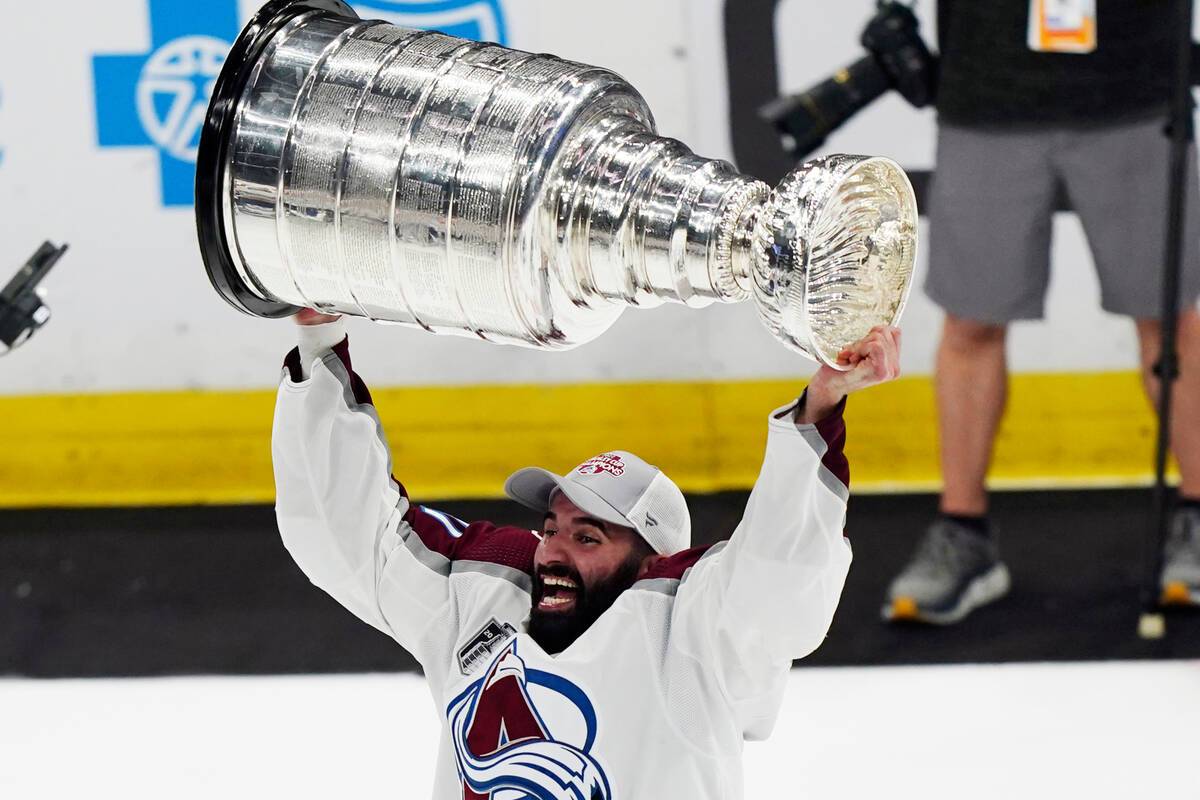In this vibrant and celebratory image, a bearded hockey player, presumably a member of the Colorado Avalanche, is captured moments after a championship victory. He stands on the ice rink, joyously holding the Stanley Cup — a massive, iconic silver trophy — high above his head. The player sports a white jersey accented with maroon on the shoulders and a distinctive maroon and blue stylized "A" logo on the chest. On his head, he wears a gray and white cap adorned with a red logo, though the specifics of the logo are indiscernible. His expression is one of sheer elation, his mouth wide open in a triumphant cheer. The background, slightly blurred, reveals a clutter of photographers, one notably dressed in a black shirt, gray shorts, and sneakers, with a large camera slung at his side. The Blue Cross Blue Shield logo is visible on the rink’s wall behind them, anchoring the scene in a recognizable professional hockey environment.